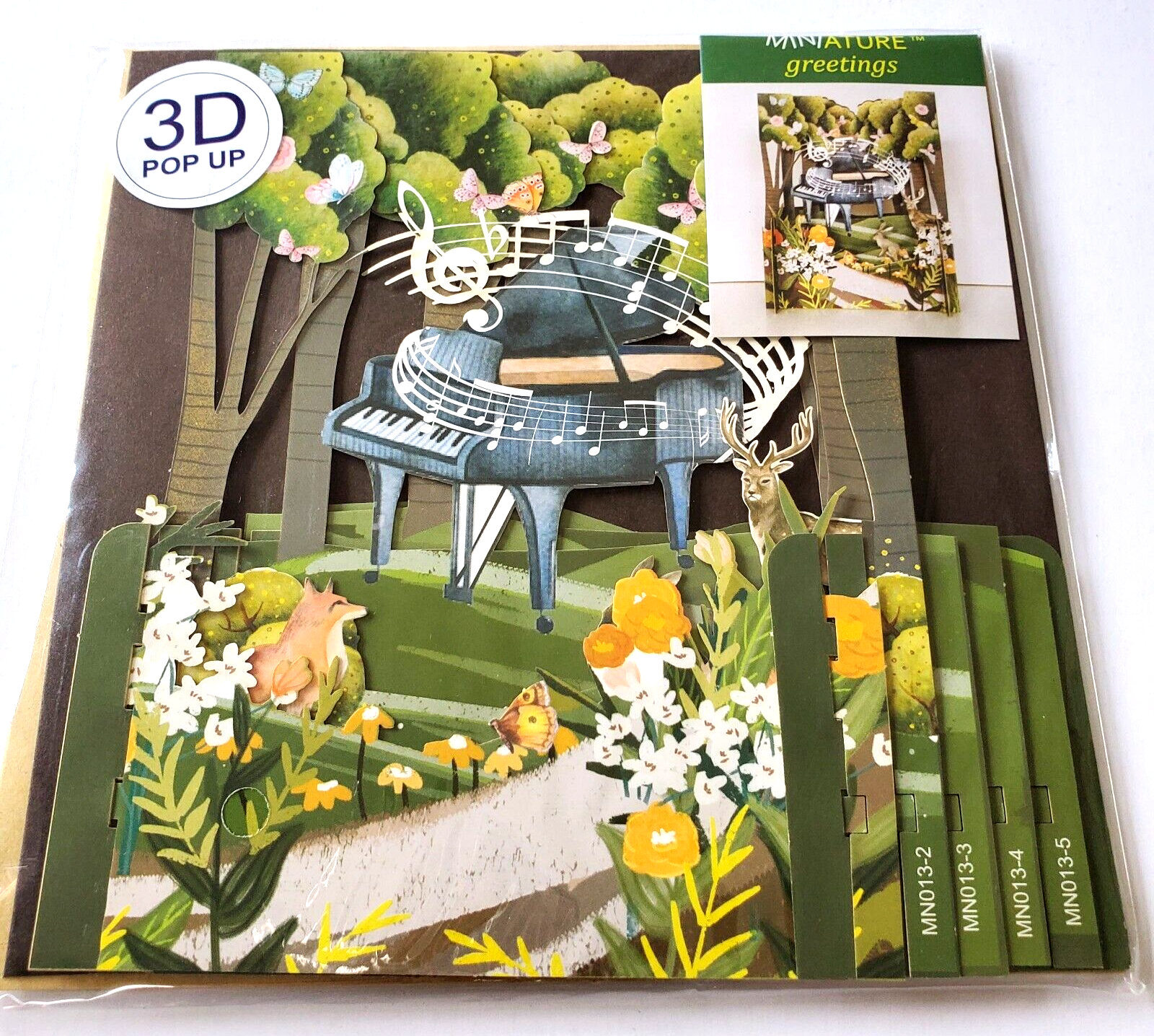This detailed image depicts the cover of a 3D pop-up book, viewed from an overhead and slight angle. The background of the cover is brown, setting a rustic tone. In the upper left corner of the cover, there is a white circle with blue letters reading "3D," and smaller black letters below that saying "pop-up." The upper right corner features a green-bordered rectangular label stating "Miniature Greetings." The centerpiece of the cover is a whimsical illustration of a black piano with white keys, blue legs, and white musical notes spiraling around it. 

In the backdrop behind the piano, vibrant green trees stretch upward, adorned with fluttering butterflies. A deer with extensive antlers faces the camera from the bottom left of the piano. Beside the deer, yellow, green, and white flowers are scattered across lush green grass. A small, brown fox is peeking up from the lower left side of the piano, surrounded by white and green plants. 

The bottom of the cover is rich with green hues, dotted with wildflowers in shades of yellow and white. Notably, small white boxes with alternating features, possibly indicating chapters, are stacked on the right, containing white lettering and situated behind a green border one-third of the way down the page. The entire cover is encapsulated in a plastic sealed bag, giving it a polished, pristine appearance.